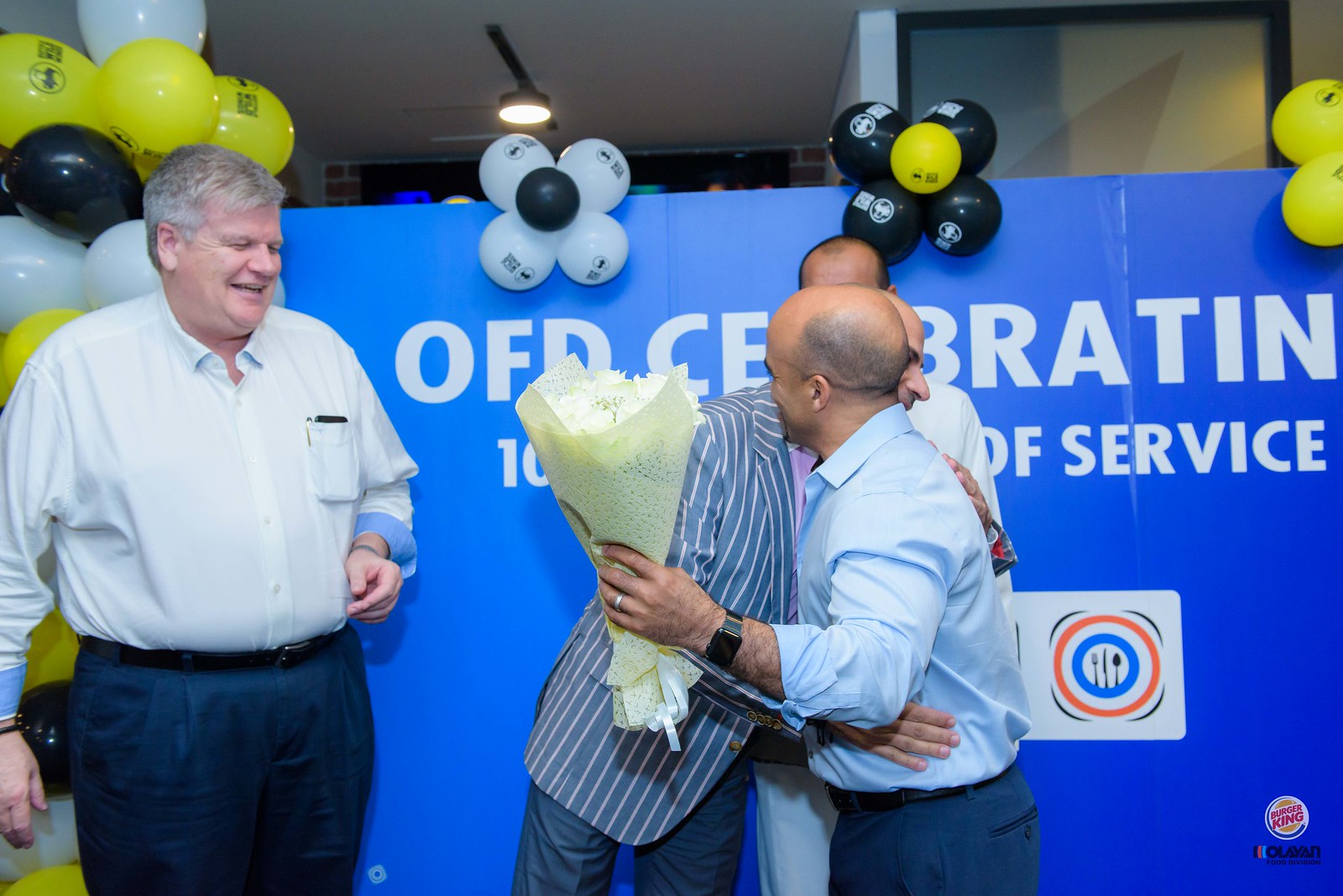In this celebratory image, three men are standing in front of a large blue banner that prominently reads "OFD celebrating" with the word "service" partially visible, hinting at a milestone—likely ten years of service. The backdrop is decorated with clusters of yellow, black, and white balloons, adding a festive touch to the scene. 

On the left side, an older man with short gray hair, dressed in a light blue button-down shirt and blue pants with a black belt, smiles warmly. He is turned at an angle towards the other two men, who are embracing in the center of the image. The man on the far right, who is also slightly balding and sporting a blue and white striped blazer over a pink shirt with blue slacks, hugs the man to his left. This middle man, also balding with a bit of facial hair, wears a light blue long-sleeved shirt, a black watch on his left wrist, and dark blue pants. He is holding a bouquet of white flowers, suggesting that he is the recipient of an award or special recognition. 

Additionally, part of a logo with an orange and blue circle featuring a fork, knife, and spoon is visible behind them, hinting that the celebration might be related to a restaurant service or hospitality award. The overall scene is one of joy and camaraderie, highlighting a moment of recognition and celebration.